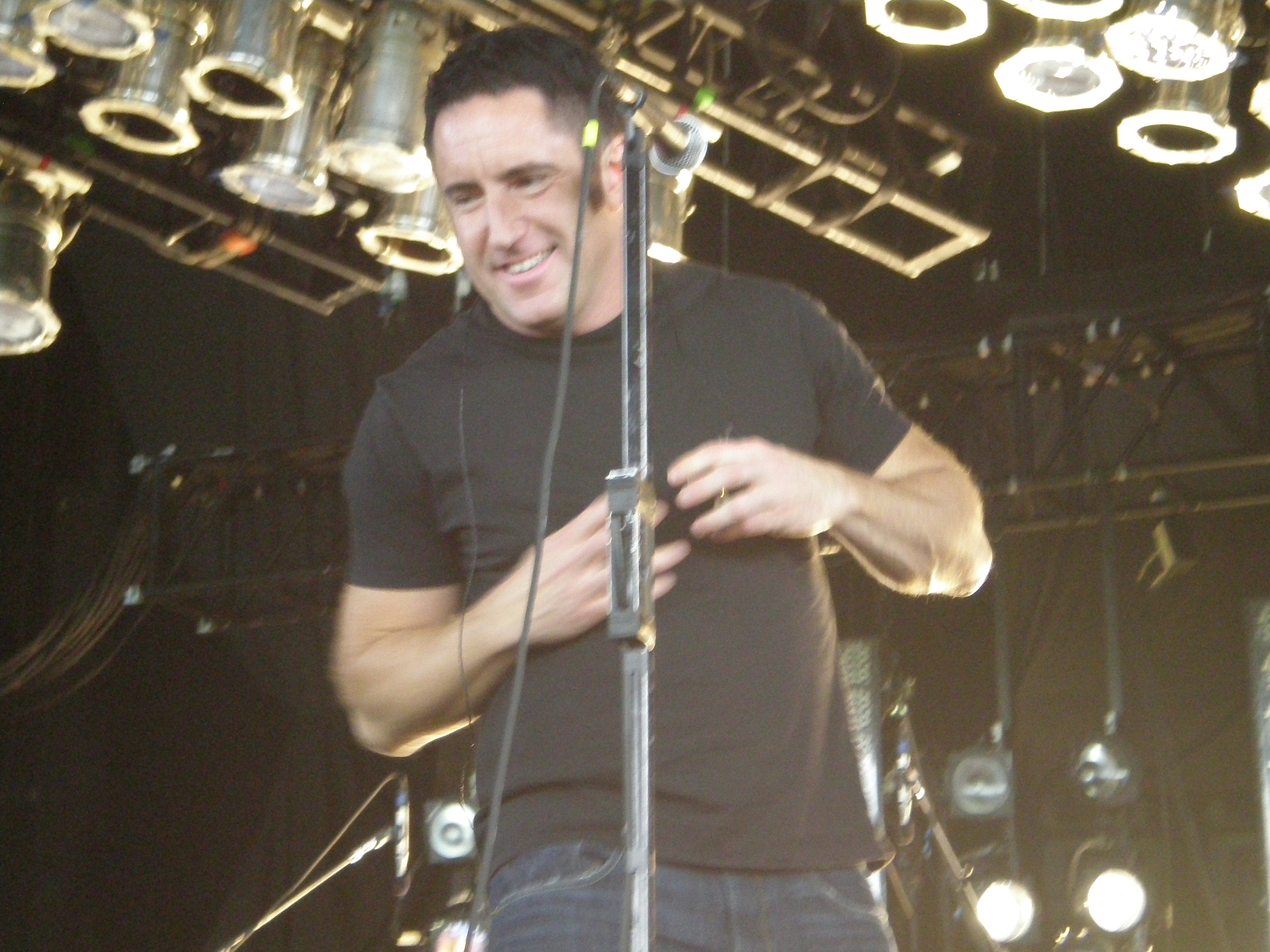This photograph captures Trent Reznor, renowned for his work with Nine Inch Nails and as an Oscar-winning composer, standing on a stage under a multitude of stage lights and spotlights, creating an atmosphere ready for a performance. He's wearing a black t-shirt and blue jeans, with a clean-shaven, short dark-haired appearance that suggests he's in his 30s. The photo, taken from a low angle, shows him from the top of his jeans upward. He is gazing down with a smile, his teeth visible, and his eyes slightly baggy. His hands are brought together near his chest, possibly holding something obscured by either his hands or the mic stand in front of him. The background is a bit dark, filled with cylindrical lights and possibly speakers, adding to the concert-like ambiance.